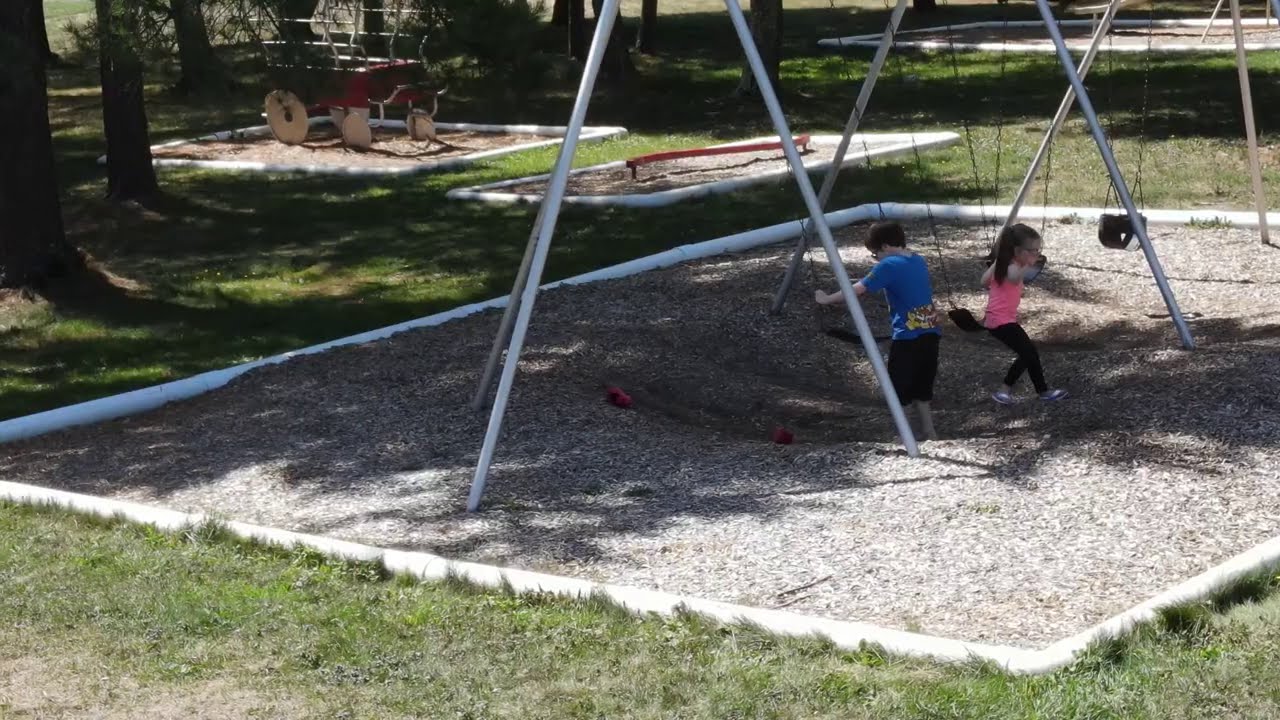The photograph captures a vibrant playground scene featuring a metal swing set with black chained swings situated on a rectangle of brown wood chips, bordered by a white PVC pipe barrier, which adds a defined structure to the area. In the center of this setup, a little boy with dark brown hair, clad in a blue shirt and black pants, stands facing away from the camera. To his right, a girl with shoulder-length brown hair, dressed in a pink tank top and black pants, appears to be jumping off her swing. The playground is surrounded by contrasting bright green grass with occasional patches of dirt.

In the background, visible on the upper left side of the image, there are additional playground areas with similar wood chip enclosures, featuring various red play structures, including a little red wagon with a barrier and a balance beam. The scenery is complemented by several tall tree trunks with hanging branches casting shadows that partially obscure parts of the grassy areas, adding depth and a natural touch to the scene.